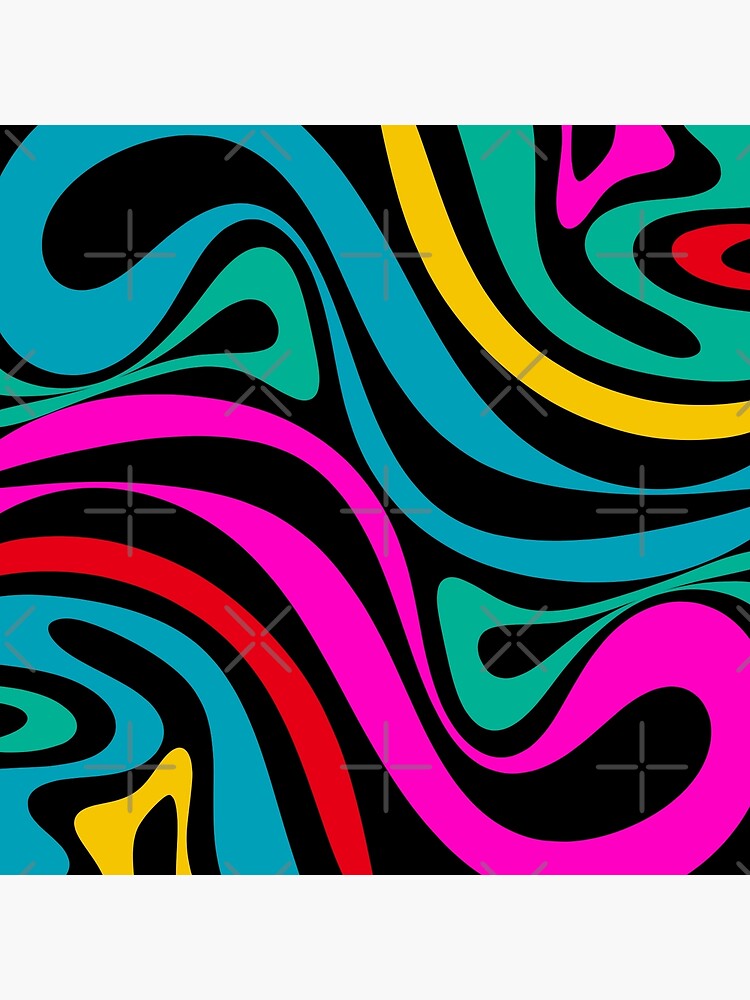The image depicts a vibrant, modern painting reminiscent of a psychedelic poster, characterized by a black background adorned with colorful swirls and lines of varying widths in a circular, intertwining motion. Prominent colors include blue, yellow, green, magenta, hot pink, red, and gold, creating a mesmerizing array of hues that seem to dance across the canvas. Subtle gray crosses divide the artwork into quadrants, adding structure and possibly serving as guides for the artist. The painting exudes a sense of fluidity and motion, captivating viewers with its intricate, swirling designs that maintain their beauty and complexity from any angle.